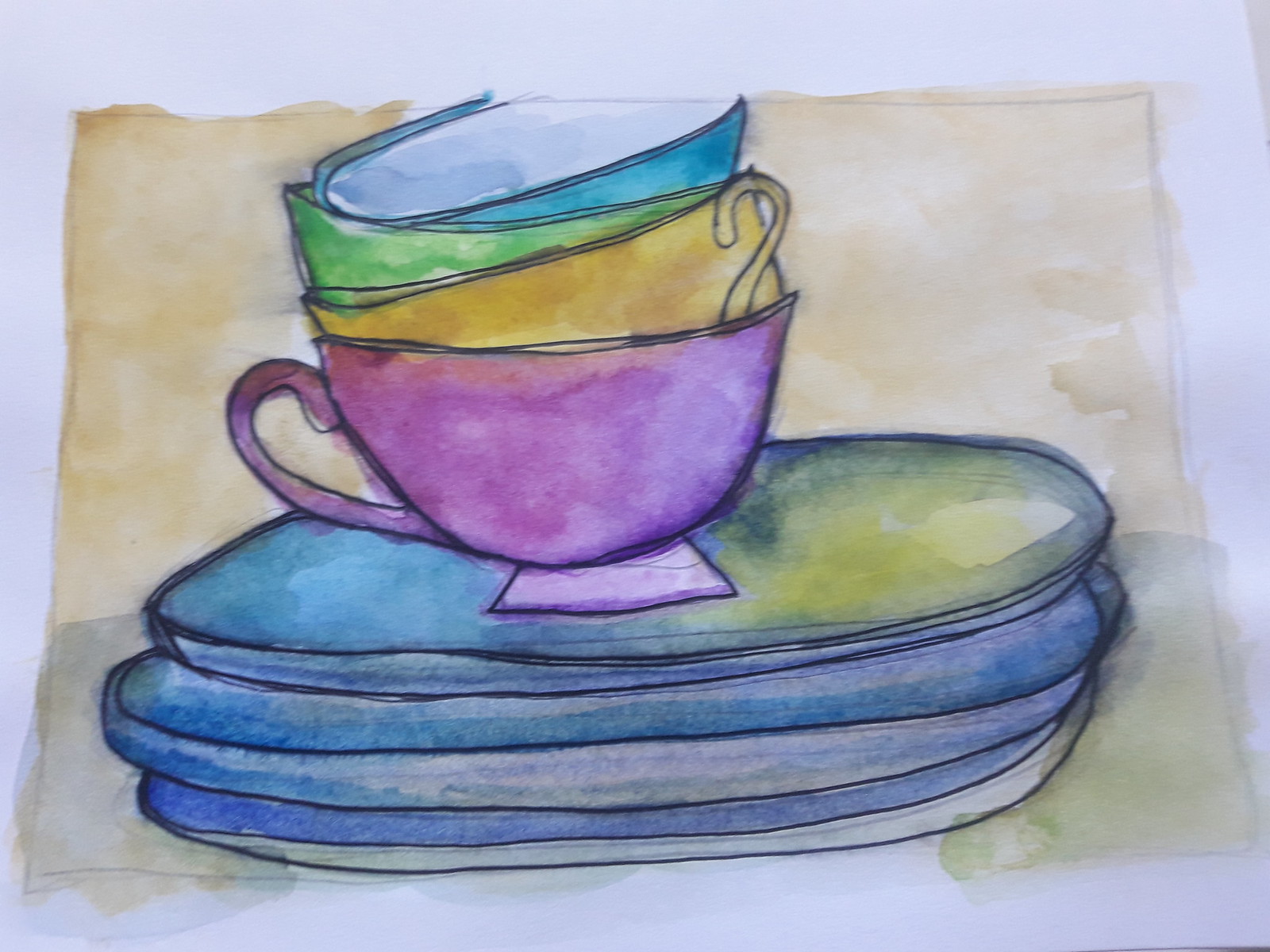A detailed watercolor painting depicts an assortment of four plates and four teacups in varying colors and arrangements. The background transitions from a light to dark yellow, adding a warm, inviting atmosphere to the composition. Each plate is primarily blue, with gradients of light blue and occasional touches of green, particularly in the top plate. The first striking teacup is a vibrant pinkish-purple, nested inside it is a yellow cup. Another teacup presents a calming green hue, while the last one is an intriguing aqua blue. The plates and cups are delicately arranged on a table, which is suggested by the white background framing the scene. This charming watercolor captures a delightful array of colors and simple yet elegant dishware, evoking a serene and homely feel.